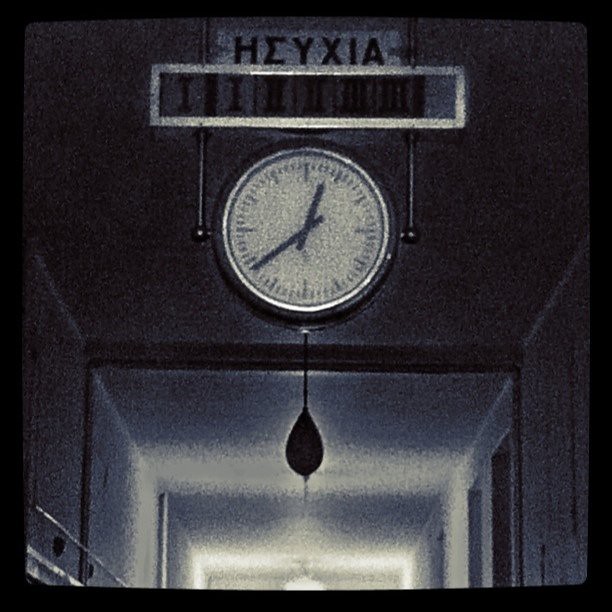A digitally altered black-and-white photograph is presented within a square frame, bordered by a rough-edged black outline with rounded corners. The image is notably pixelated, giving it a mosaic-like texture of thousands of tiny dots. The scene within the frame depicts a slightly surreal corridor. Dominating the upper center of the image is a white rectangular sign bearing text in Greek. Below this, attached by two slender metal arms, hangs a large circular clock. The clock face is minimalist, marked only with extended lines at the 12, 3, 6, and 9 positions, and shorter lines demarcating the other hours. The time displayed is 12:34, with the clock hands represented as sleek, elongated ovals. Situated beneath the clock is a dark, almost indistinguishable object that vaguely resembles a punching bag, though it seems out of place in the corridor setting. This curious composition is punctuated by a single, intense light source at the bottom center, casting a bright glow and drawing the viewer’s attention to the otherwise dimly lit surroundings.